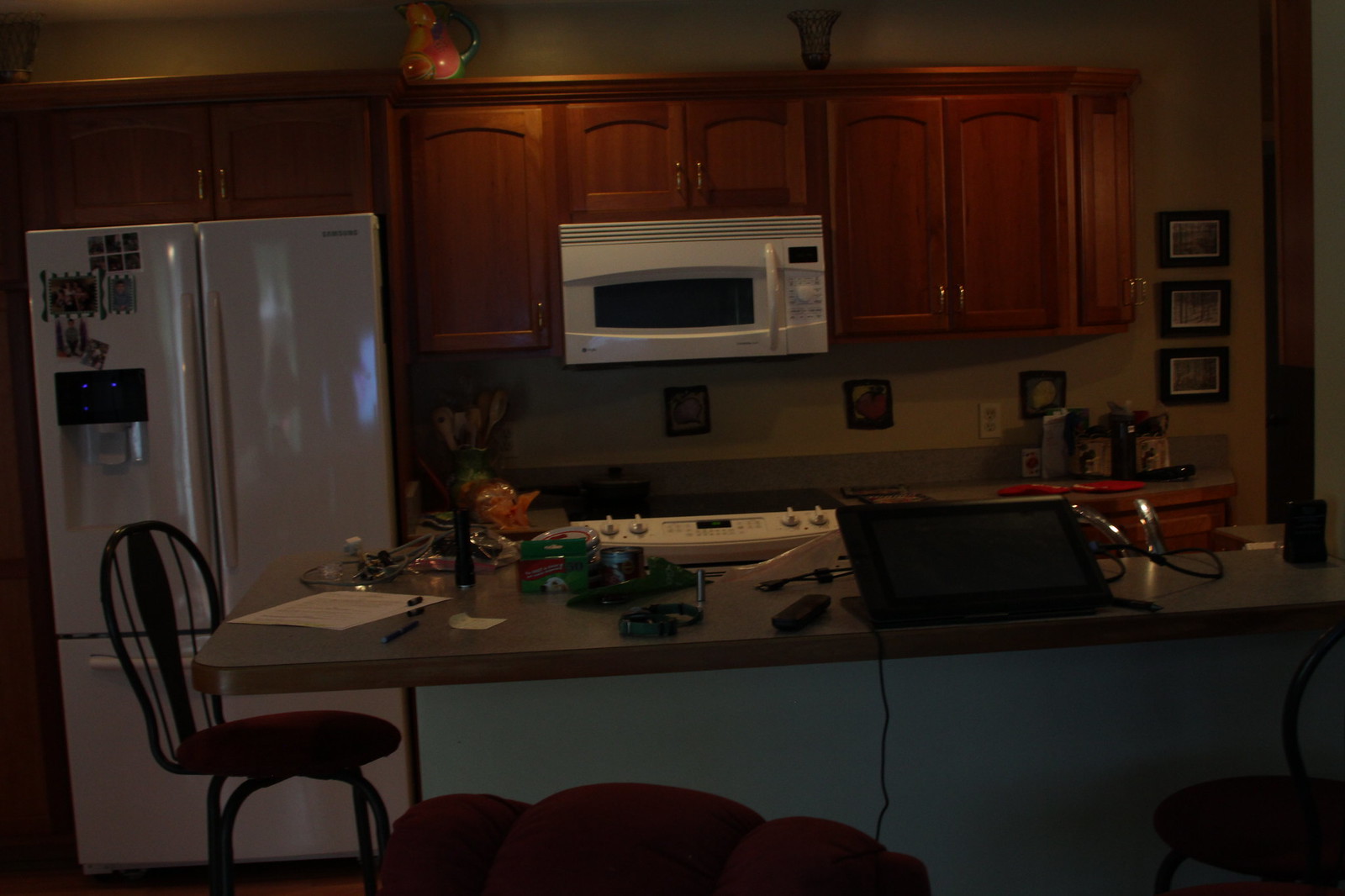The image depicts a modern kitchen setting, rich in detail and color variation. At the bottom of the image, there's a partial view of a dark purple chair. To the right, there is a black chair, while to the left, there is another black chair featuring a brown circular cushion. Central to the scene is a countertop with a base in light gray and a rectangular tabletop in a brownish-gray hue. On this tabletop, prominently displayed, is a black iPad and a small black remote situated to its left. Further along to the left, a vertical black flashlight is standing up beside a collection of green objects.

In the background, the left side of the image features a light gray refrigerator. Above the refrigerator, a series of brown cabinets line the wall, with a white microwave nestled beneath them. The microwave has a white handle and a set of buttons on its right side. Underneath this arrangement, a series of small, square, black-framed pictures are displayed on a light tan-colored wall, adding a touch of personal decor to the setting. The overall composition offers an inviting glimpse into a contemporary and well-appointed kitchen.